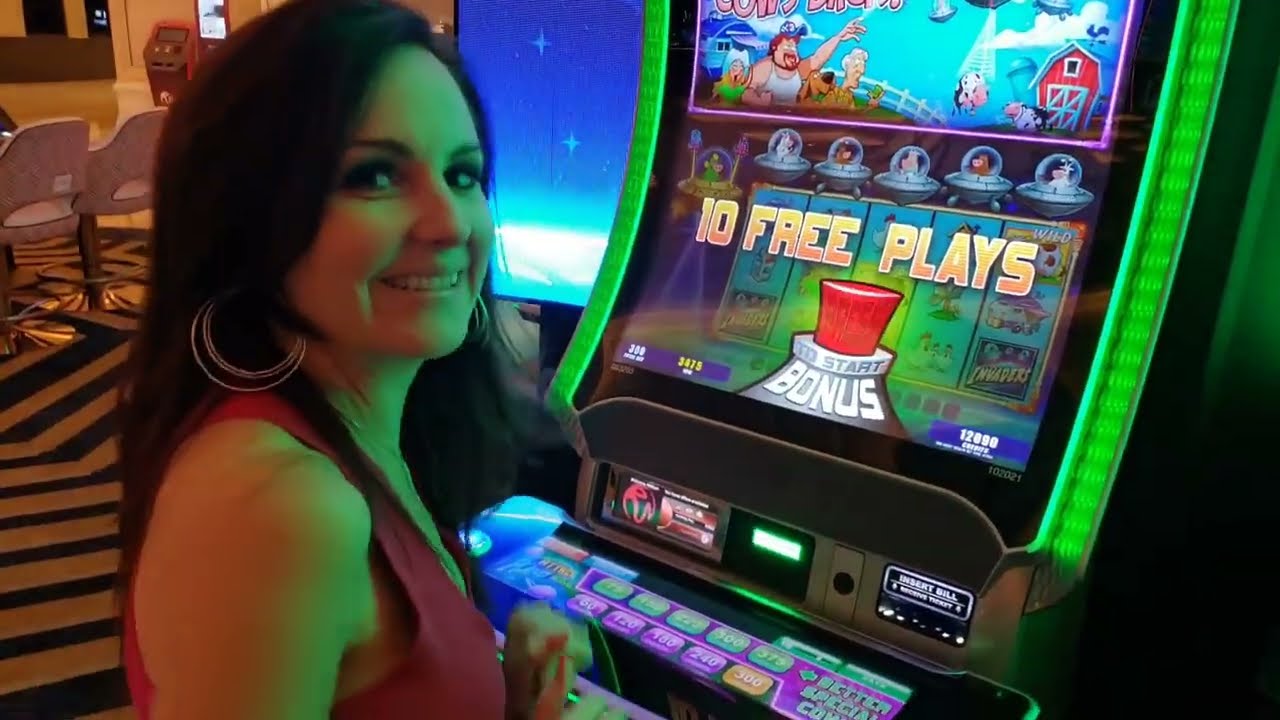In the image, a young woman with long black hair and large silver hoop earrings, comprised of multiple smaller hoops, stands while engaging with a brightly lit slot machine in a casino. She wears a pink tank top with short sleeves and is smiling warmly towards the camera. The slot machine in front of her is adorned with various colorful and lively graphics, including cartoon-like characters, a red barn, a blue sky, and a white picket fence. 

The machine prominently displays "10 Free Plays" in yellow letters and has a red button labeled "Bonus" with green lighting around its perimeter. Above the screen on the machine, there are images of farm animals, including a cow, a pig, and a wolf, as well as people in different outfits, including a woman in a green shirt and a man in a white tank top and blue hat.

Buttons on the slot machine show different betting options with amounts in vibrant colors like purple and orange, ranging from 180 to 540. The background of the scene features white chairs facing away from the machine and a carpet with black and gold stripes. The setting inside the casino is illuminated with various other machines and a tan-colored wall, contributing to a busy, vibrant atmosphere.